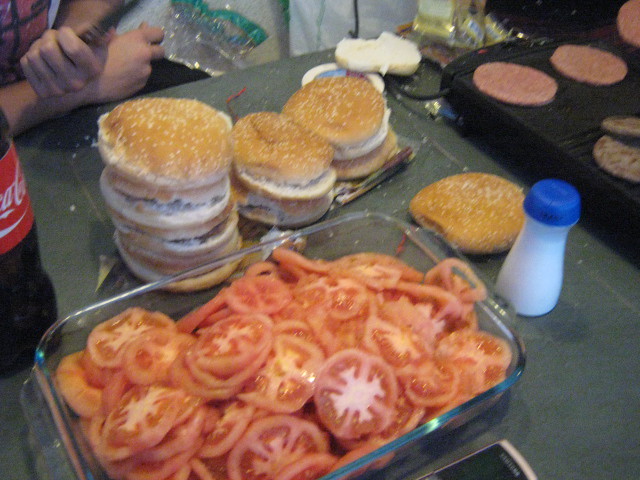The photograph appears to be of a casual dining setup, possibly on a porch or patio, featuring a table filled with the makings for hamburgers. The image is somewhat blurry and pixelated, likely taken with a phone or older digital camera. Centered in the foreground is a large, rounded rectangle glass casserole dish filled to the brim with neatly sliced ripe red tomatoes, resting on a gray tabletop. Just behind this glass container, there are several sesame seed hamburger buns arranged in three stacks: a tall stack of approximately eight buns on the left, and two shorter stacks of three to four buns each, alongside a single bun off to the side.

To the left of the glass dish, part of a Coca-Cola bottle with a distinctive red label is visible, though its size is indeterminate. On the right side of the table, slightly behind the tomato slices, stands a white bottle with a blue cap, lacking any label to identify its contents, which could possibly be mayonnaise. 

In the upper left corner of the frame, a person with tan or light brown skin is visible, though only their hands and a section of their red shirt with black details can be seen as they hold something out of focus. 

Dominating the upper right corner of the image is a small, simple grill. It bears several hamburger patties in different stages of cooking; uncooked patties occupy the left side, while the right side shows patties that are cooked to varying degrees. The setting suggests a laid-back and communal meal, with all elements prepared and ready for assembling into delicious hamburgers.